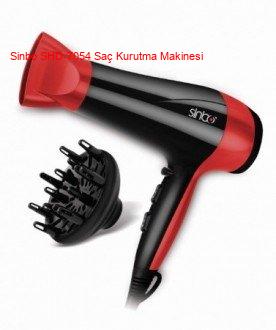This image depicts a European-style hair dryer floating against a white background, exhibiting a striking black and red color scheme. The main body of the hair dryer is black with a distinct red stripe running along its length, accentuated by a small black section at the end. The barrel tapers into a thinner part designed to focus the airflow. The brand name "Sinbow" is prominently displayed in white text on the device, though there's additional text that remains too blurry to read. The controls are situated on the black portion of the dryer. Attached to the nozzle is a red diffuser, which appears detachable. To the side of the hair dryer lies an accessory, resembling a scalp massager. The power cord can be seen extending from the bottom, gradually disappearing into the white background.